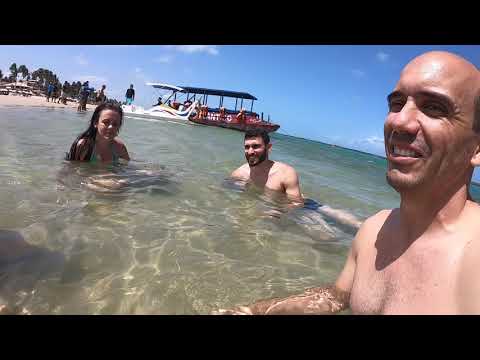The image is a wide rectangular photograph featuring three people swimming in shallow ocean water near a beach under a mostly clear blue sky with some white clouds. The beach, located on what seems to be an island, has green trees in the background and is populated by several people walking or standing near tables with umbrellas. In the foreground, on the right, is a smiling bald man, while in the middle is a man with brown hair and a beard, leaning to his right. To their left is a woman in a bikini, submerged up to her shoulders, with long dark hair. Behind them floats a long red ferry boat with a roof, and a small white boat with a roof is also visible further in the background. The horizon line starts at the top left and slopes downwards towards the middle right of the photo. The image is framed by black stripes at the top and bottom, giving it a cropped appearance. It is taken during the daytime.